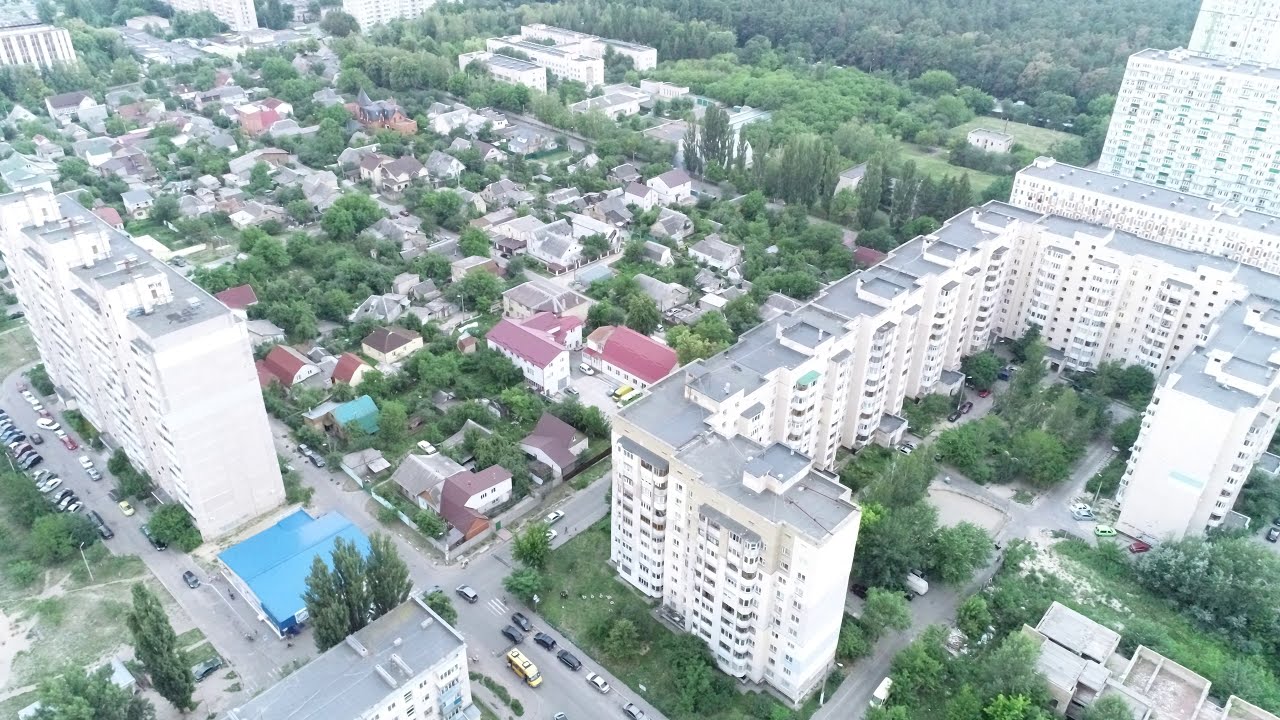The image provides an aerial view of a residential area within a city. Prominently featured are two large, white apartment complexes: one on the left side of the image with a boxy, rectangular shape, and another on the right, which has a distinct U-shape. Both buildings are multi-leveled and adorned with numerous windows and balconies. Between these towering structures lies a neighborhood of shorter, traditional houses with roofs in shades of red, brown, and gray. Streets crisscross the scene, populated with a variety of cars in colors including black, yellow, red, and blue. Trees are scattered throughout, adding pockets of greenery, with a denser section of tall trees visible towards the top of the image. The composition highlights a diverse and dynamic urban landscape, absent of people or text.